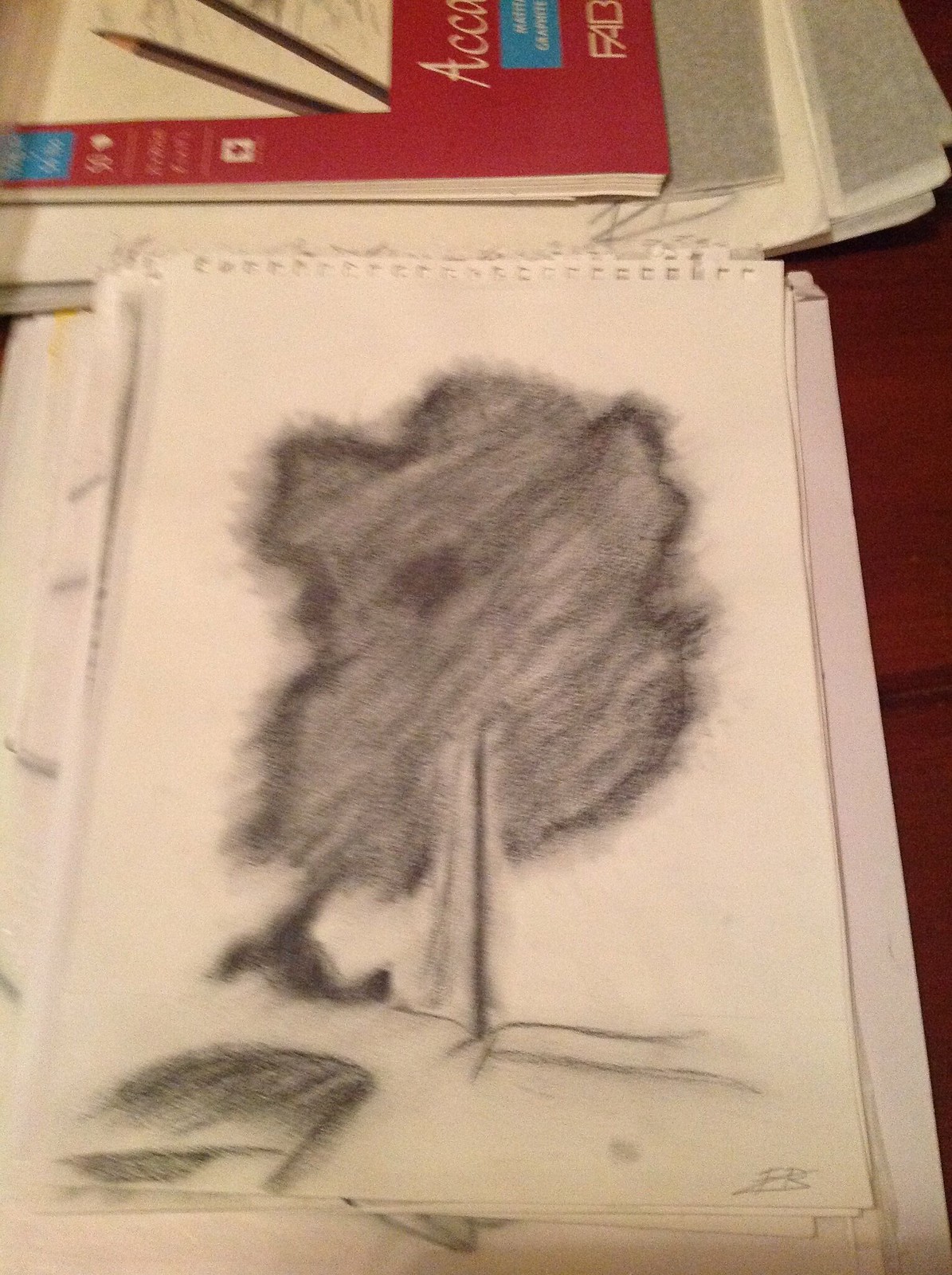A sheet of paper, appearing to be torn from a notepad, sits on a medium dark brown wooden table. The top edge of the paper is lined with numerous tiny square holes, indicating it was ripped out of a spiral-bound notebook. In the background, a red book is partially visible. The focal point of the paper is a pencil sketch, depicting a tree with intricate branches and foliage. Beneath the tree, a small figure can be seen—potentially a person, bird, or some other animal. At the base of the sketch, there's a delicate drawing of a flower and a leaf. The artwork is signed with the initials "eb" at the bottom left corner.